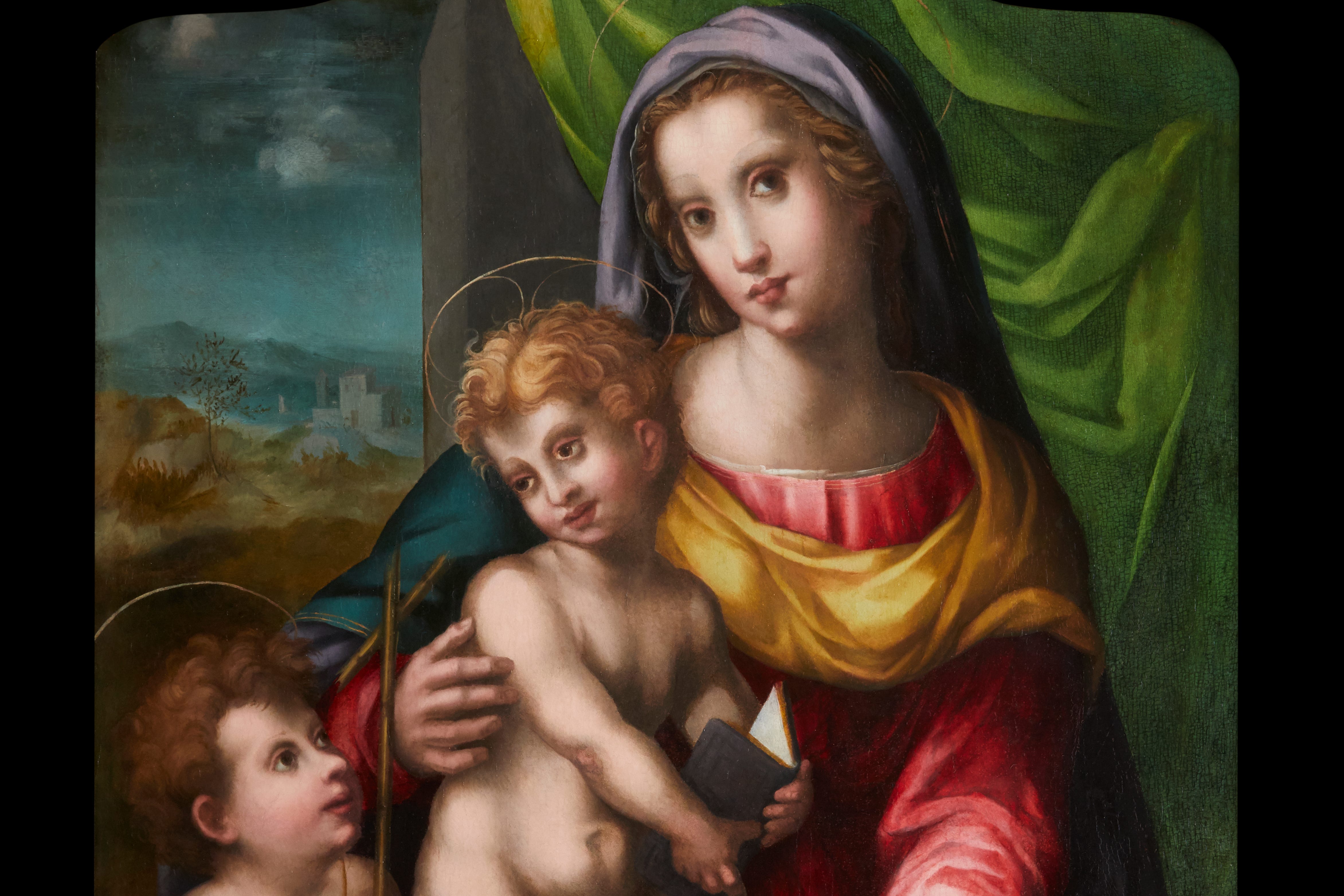The image is an oil painting depicting a serene Madonna with two nude children, possibly cherubs, nestled against her. The Madonna, a white woman with soft brown hair, dons a black and grey veil over her head, accompanied by a yellow shawl draped over a red dress. Her head tilts gracefully to the side as she gazes directly ahead, with a nurturing arm around one of the children. The child in her arms, looking away from her, and the other child, gazing up at her from the bottom left, both have halos around their heads. The children's hair, one blonde and the other brown, appears soft and delicate. They sit on her lap, basking in the serene ambiance created by the scene. Behind them, a green curtain frames the backdrop, giving way to a grey wall and a distant landscape with a sky adorned with clouds, transitioning to blue, and a vast mountain range over brown, earthen terrain. The painting evokes a traditional Madonna and Child composition, rich in religious symbolism.